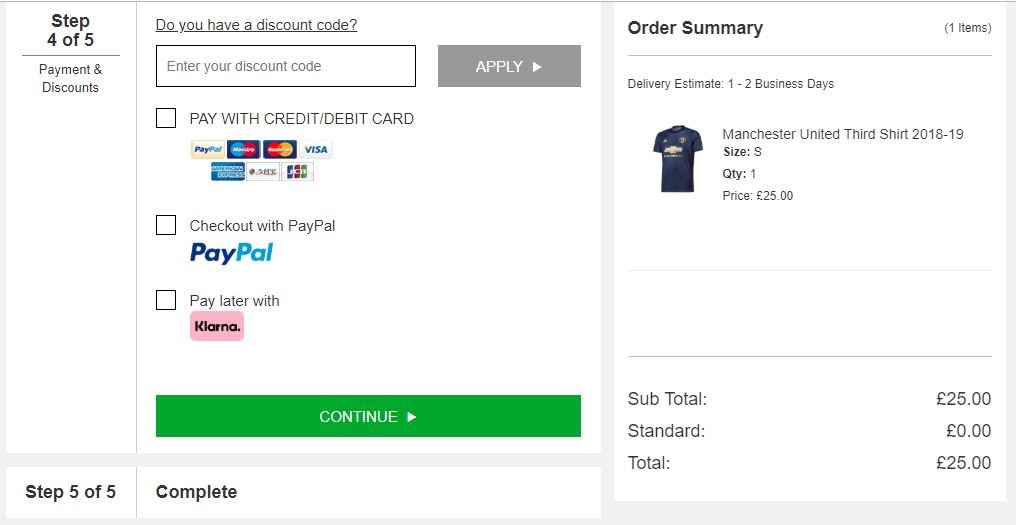This image captures a detailed view of an order summary page on an e-commerce site. Starting from the top left corner, the page indicates, in black text, that the user is on step four of five. Below this section, there's a horizontal line separating it from the "Payment and Discounts" section. At the bottom of the left side, there's another indicator showing step five of five.

In the middle of the image, there's a prominent section asking, "Do you have a discount code?" with a text box underneath for entering the code. Next to the text box, there is a button labeled "Apply." Below this area are various payment options including "Credit Card," "Debit Card," "Checkout with PayPal," and "Pay Later with KLARNA," each accompanied by their respective logos. Under these options is a green button labeled "Continue," followed by the word "Complete."

The right side of the image features the order summary. At the top, "Order Summary" is displayed in black text, followed by a delivery estimate of one to two business days. Below this, product details are listed: a Manchester United T-shirt from the 2018-2019 season, size small, quantity one, priced at £25. The subtotal is £25, with standard shipping listed as £0, bringing the total to £25.